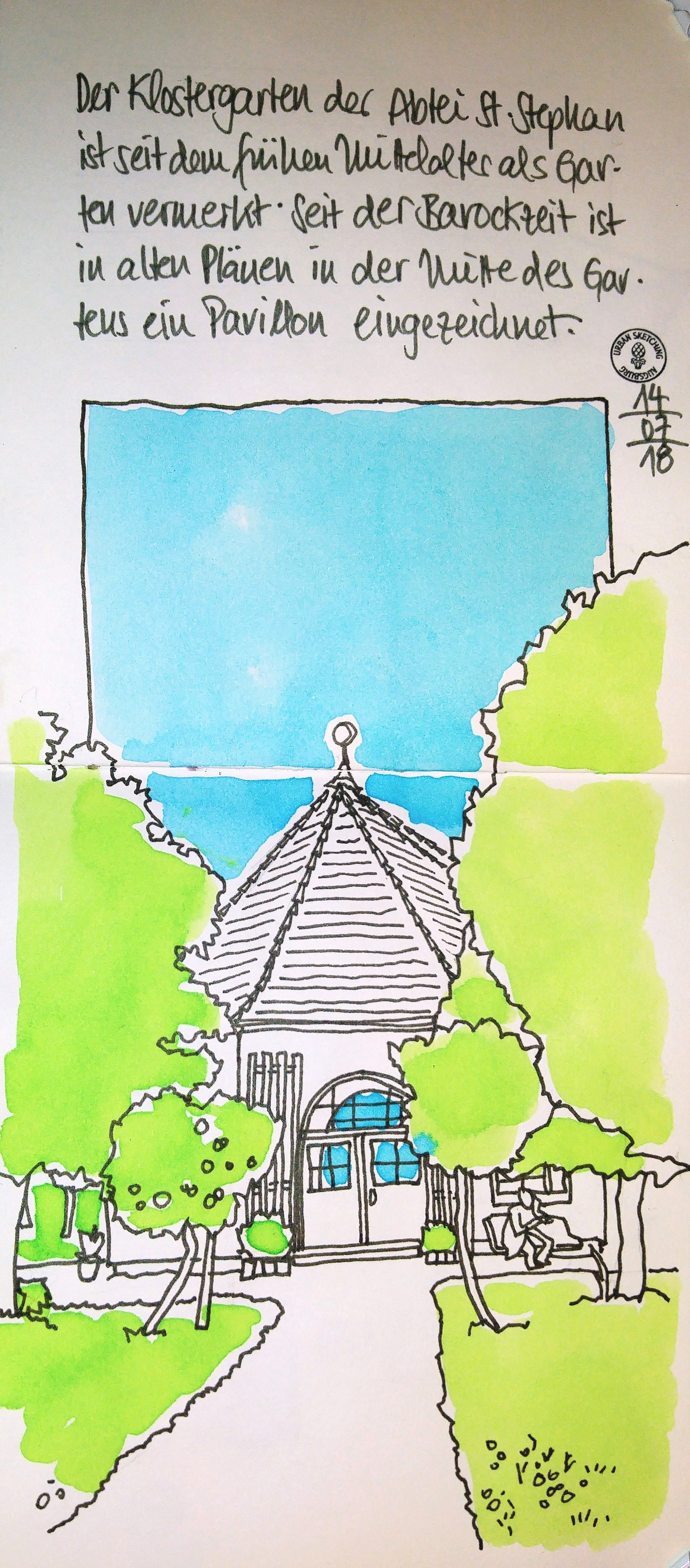The illustration depicts a charming building with a strikingly picturesque blue sky as its backdrop. At the top of the image, there is black script, presumably written in a language that appears to be German or Dutch. This writing overlays a bright blue, rectangular expanse of sky, which gracefully descends and is interrupted by the pointed structure of the building’s rooftop.

The building itself boasts white walls and a distinctly triangular, white roof accentuated with black horizontal lines, giving it a classic, structured appearance. Flanking the building on either side are lush green patches of grass, each adorned with verdant trees showcasing dense, leafy canopies.

In the foreground, just to the right of the two white doors that lead into the building, a person is seen sitting on a bench, adding a touch of human presence to the serene and verdant scene. The intricate details and vibrant colors of this drawing bring a sense of tranquility and charm.